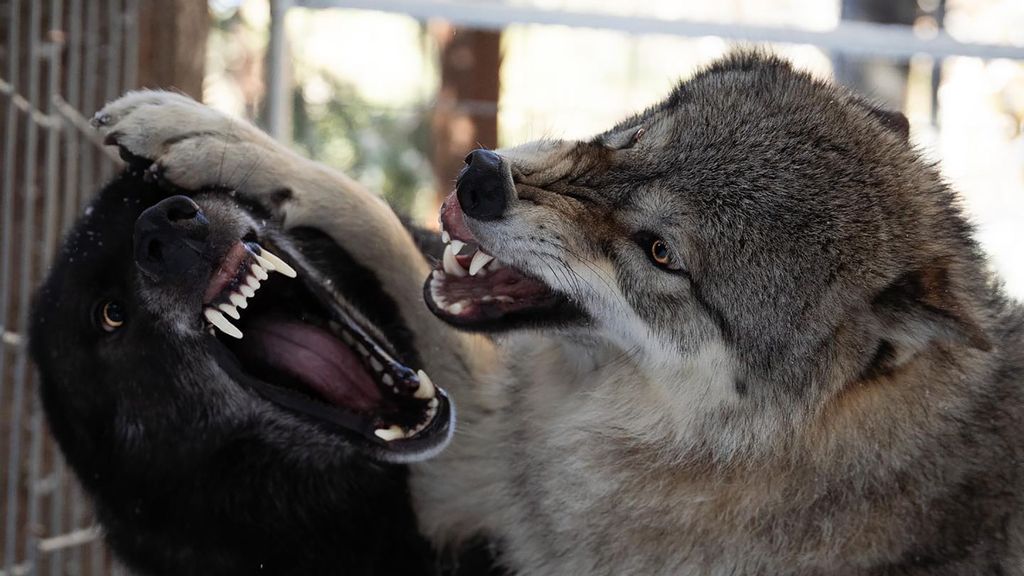In this outdoor image, two fierce-looking dogs, possibly wolf hybrids, appear to be engaged in a serious fight within a gated area. The dog on the right, which resembles a husky with traditional wolf coloring, has a gray head, white around its mouth, and brownish fur mingled with the gray and white. This dog is snarling, its face scrunched up, with one paw pressing down on the head of the black dog to its left. The black dog’s mouth is wide open, baring its teeth and showing a hint of white around its mouth. Both animals have striking pale yellow eyes. The close-up shot captures their intense expressions and open mouths, highlighting their aggressive stance. The background features a fence to the left, along with some indistinct buildings or structures and barely visible trees, hinting they are within a controlled environment.